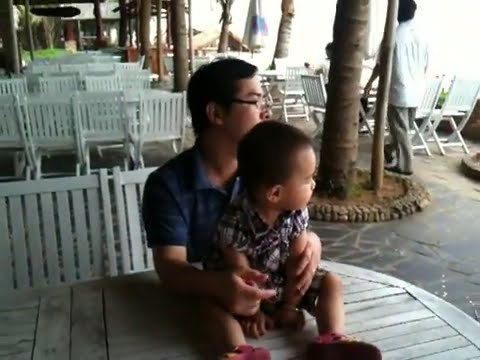In this outdoor photo, a glasses-wearing Asian man is seated on a white wooden chair at a table, holding a toddler child who is sitting directly on the table. The man is clad in a Doc t-shirt, and the child wears a black and white shirt along with red sandals. Surrounding them, the area features rows of similar white chairs and brownish-tan tables, suggesting a business or patio setting. In the background, multiple tree trunks are visible, and to the right, a prominent tree trunk stands near the man and child. Additionally, another man in a white shirt and gray pants is walking away from the seated pair, further punctuating the scene. The floor consists of gray stone, and the overall sky is gray, indicating an overcast day. The presence of umbrellas on some tables and the beach-like ambiance adds character to the serene, communal environment.